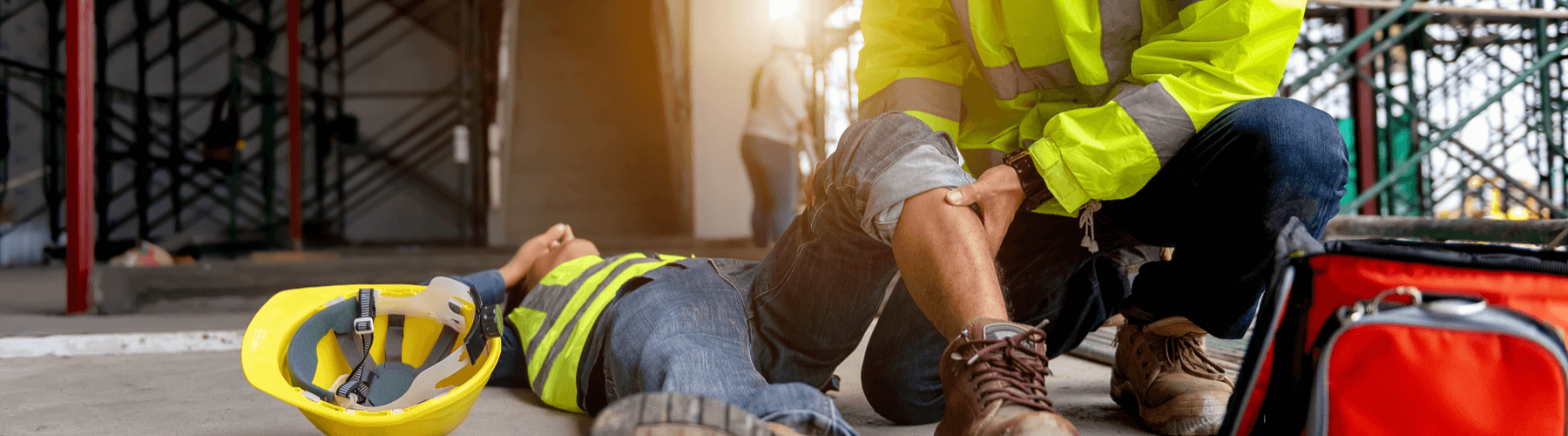The image depicts a construction site scene, possibly indoors, surrounded by exposed walls, girders, and beams. Central to the image, a construction worker lies on his back on the ground, his left leg bent upwards and his right hand on his face, suggesting he is in pain. He is dressed in blue jeans, brown shoes, and a fluorescent yellow safety jacket. His yellow hardhat with gray straps is positioned to his right. Another worker, identifiable only from the lower abdomen down, is squatting beside him. This helper is also wearing blue jeans, brown shoes, and a yellow safety jacket, and is closely examining the injured man's bent leg, which has the jeans rolled up to expose the knee. In the bottom right corner, a bright red canvas bag, likely a first aid kit, is visible. The background is filled with scaffolding and construction materials, emphasizing the active work environment. Additionally, a third worker can be seen in the middle back of the image, engaged in his tasks. The scene captures a moment of injury and immediate assistance amid a bustling construction site.